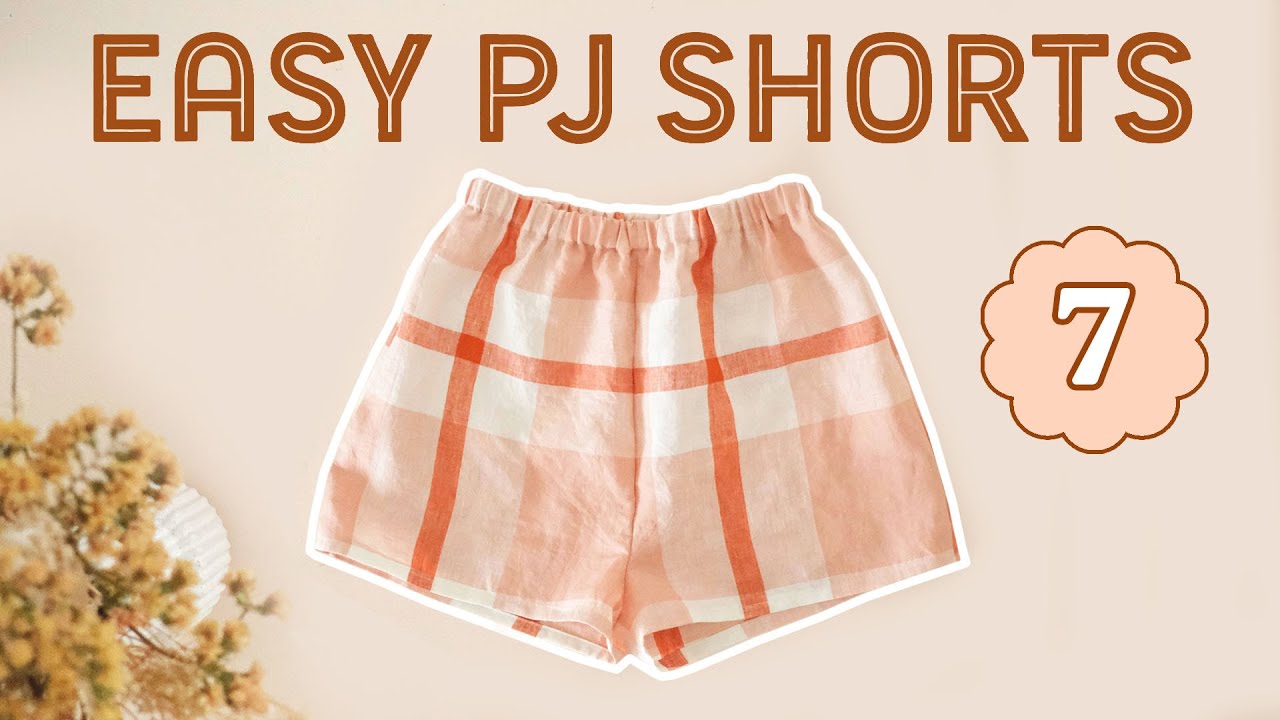This image is a detailed advertisement for women's pajama shorts set against a light beige background. Prominently displayed in the center are thigh-high pajama shorts featuring a soft plaid pattern in peach, coral, and white colors with red stripes running horizontally and vertically. Above the shorts, in bold brown capital letters, the text reads "Easy PJ Shorts." To the right of the shorts, an illustrated pink cloud with a brown outline encases the white number 7. On the left side, there is a potted plant with yellow flowers in a white container, which also seems to contain a seashell. The background complements the overall aesthetic with a very light peach hue, evoking a calm and inviting feel typical of a catalog display.